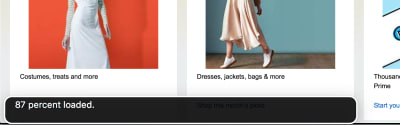The image appears to be a partial screenshot of a retail webpage focused on dresses. The visible portion showcases two promotional images of women in dresses, both of which are partially cropped.

On the left side, a woman is dressed in a white gown reminiscent of a wedding dress, set against an orange background. The image is cut off just above her chest, leaving the upper portion of her body out of view. Beneath this image, there is text that reads, "costumes, treats, and more."

On the right side, another image features a woman in profile, facing left. She appears to be on tiptoes or taking a step up, revealing her bare legs and white shoes. She is dressed in a beige or tan skirt, and the image is cropped at the waist. The background features a blue wall and a brown floor. Below this image, the text states, "dresses, jackets, bags, and more."

At the bottom of the image, there is a prominent black bar with white text indicating "87% loaded." Additionally, a small portion of another image can be seen on the far right, displaying blue and white colors.